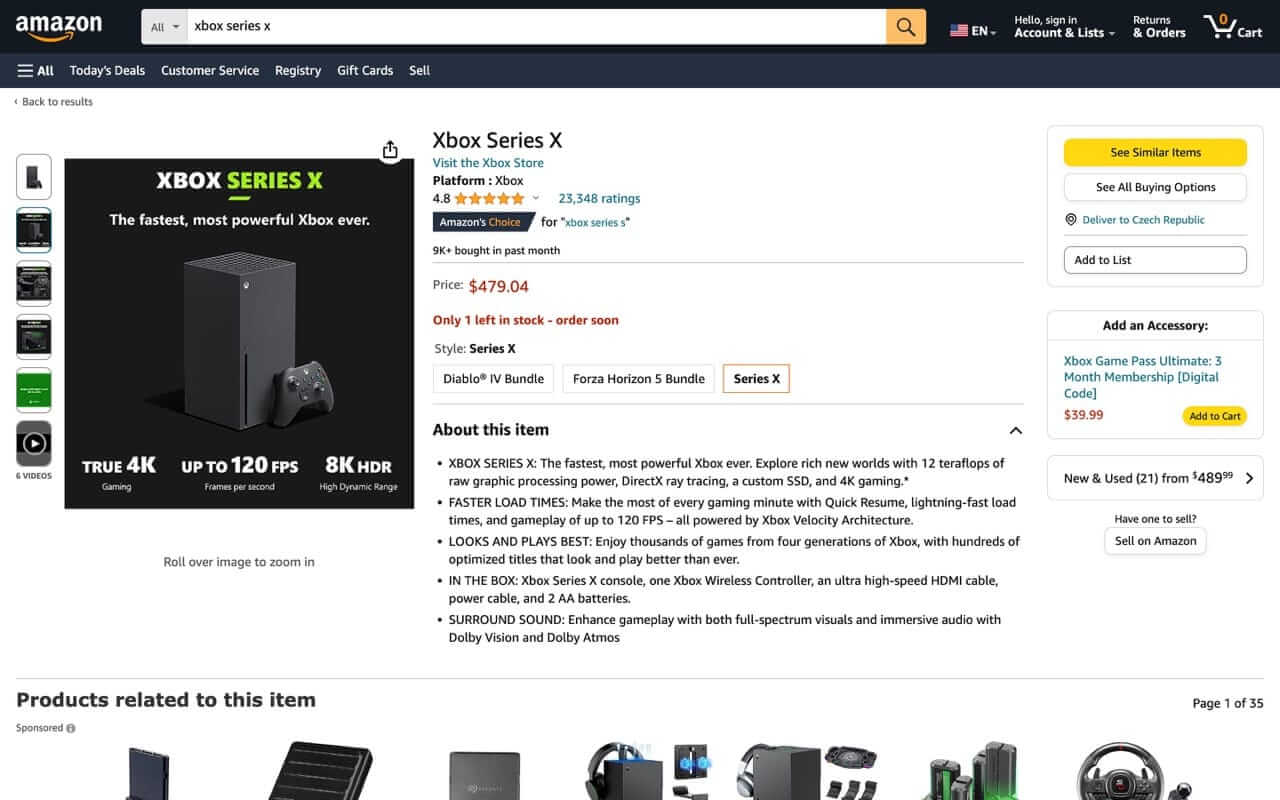The image displays an Amazon product page for the Xbox Series X. The search bar at the top includes the text "Xbox Series X," and below it are links for "Today's Deals," "Customer Service," "Registry," "Gift Cards," and "Sell." Dominating the center is a prominent black box with text proclaiming the Xbox Series X as "the fastest, most powerful Xbox ever." 

The product image showcases a sleek, gray, cube-like Xbox Series X console, accompanied by a controller positioned to its right. To the left of this image, promotional text highlights its capabilities, stating "True 4K up to 120 FPS" and "8K HDR."

Further details specify: "Xbox Series X, Visit the Xbox Store," the platform being Xbox, and a stellar rating of 4.8 stars from 23,348 reviews. It's designated an "Amazon Choice for Xbox Series X," with over 9,000 units purchased in the past month. The listed price is $479.04, with a critical note that only one item is left in stock, urging potential buyers to "order soon."

Additionally, the product style is identified as "Series X Diablo 4 Bundle for the Horton 5 Bundle Series X." The section ends with a prompt to learn "about this item," suggesting further detailed information is available.